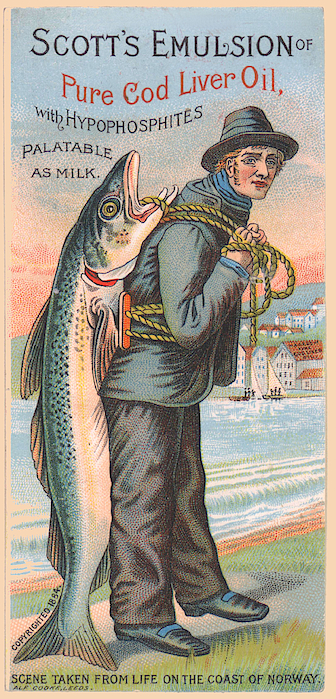The image, a tall and narrow vintage advertisement, depicts a cartoonish scene promoting "Scott's Emulsion of Pure Cod Liver Oil with Hypophosphites Palatable as Milk." The central figure is a man outfitted in a gray jacket, brown pants, and a black hat, though other accounts suggest he might also be wearing a blue scarf and black leather shoes or a blue hat and blue shoes. The man is slightly leaning to the right and firmly grasping a rope that secures an enormous fish to his back. The fish, nearly as tall as the man, has its mouth open with the rope encircling its bottom jaw. The back of the fish is portrayed as blue with gray fins and a white belly. In the backdrop, an expansive ocean wave rolls in front of a small coastal village characterized by buildings with orange roofs. The scene, captioned "Seen taken from life on the coast of Norway," suggests authenticity and is further contextualized by the image's claim of being copyrighted in 1854.